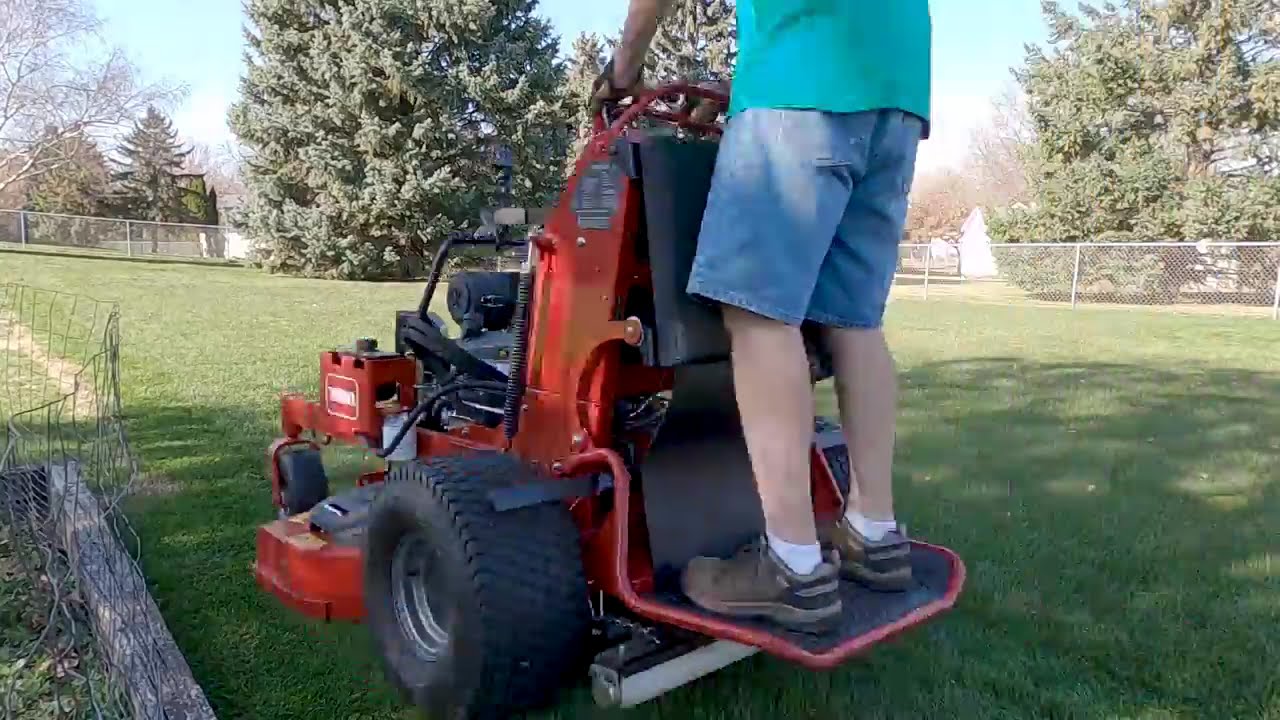In a spacious, well-maintained backyard with neatly trimmed grass, a commercial Toro lawnmower with a copper-red body and the word "Toro" printed in a white font on the front is being operated. The lawnmower features two large rear wheels and two smaller, swivel front wheels. A person stands on a small black platform at the back, steering the mower. They are wearing brown and gray shoes, white ankle socks, blue denim shorts, a teal shirt, and light brown gloves. Their legs are exposed from the knees down, and they are gripping the mower's handlebar. In the background, a chain-link fence encloses the area, accompanied by several tall evergreen trees and a leafless deciduous tree. The sky is a clear, vibrant blue. A bundle of wire on a piece of wood is visible in the bottom left corner of the image.